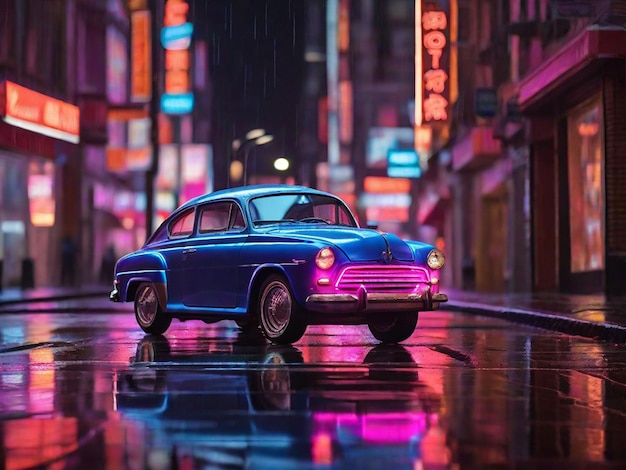In the image, a classic royal blue coupe from the late 1950s or early 1960s is prominently featured on a wet city street at night. The car, likely of Japanese make, is a two-door model adorned with more chrome than contemporary vehicles, showcasing a vintage aesthetic typical of that era. The coupe is angled with its front pointing towards the bottom right of the image, displaying its pinkish-purple grill and twin round headlights. The urban backdrop is vibrant with illuminated high-rise buildings and blurry neon signs bearing Japanese characters, intensifying the car’s old-fashioned charm. The street, glistening from recent rainfall, and the myriad of city lights contribute to the artistic and nostalgic atmosphere of the scene, suggesting it is a modern photograph of a classic vehicle, potentially a highly detailed replica.